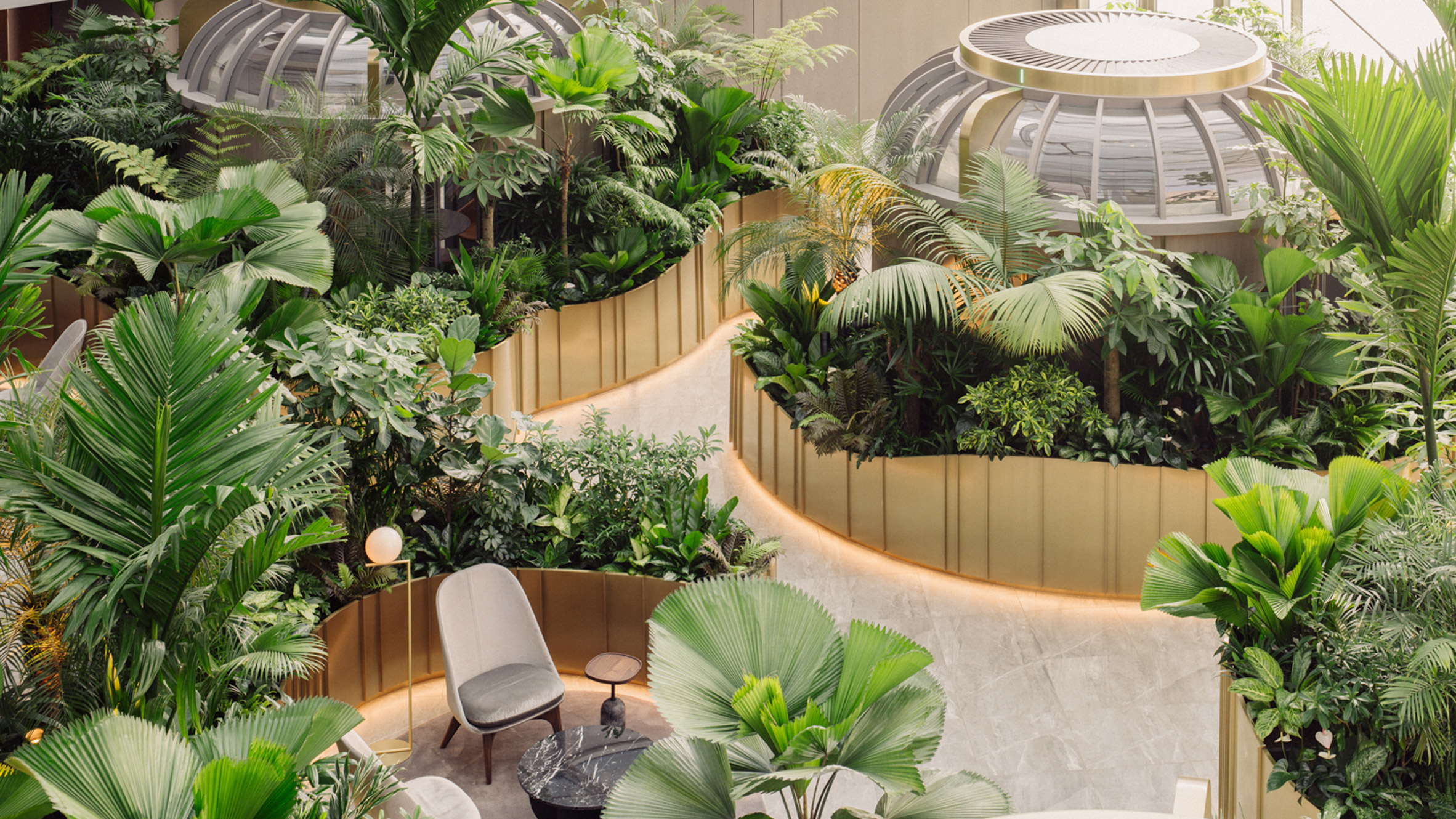The image presents a detailed, computer-generated concept of a lush, indoor botanical garden featuring two prominent greenhouse-like domes. These structures, enclosed with glass or plastic, are surrounded by verdant vegetation including ferns, tropical palm trees, and a variety of other plants. Interspersed among the greenery are small lounge areas furnished with chairs and end tables, creating intimate meeting pods or relaxation spaces. Walkways, possibly made of concrete, weave through the dense foliage, illuminated subtly where brass-like walls meet the ground, enhancing the serene environment. The overall setting appears to be part of an elaborate interior design integrating nature seamlessly with functional meeting and leisure spaces.